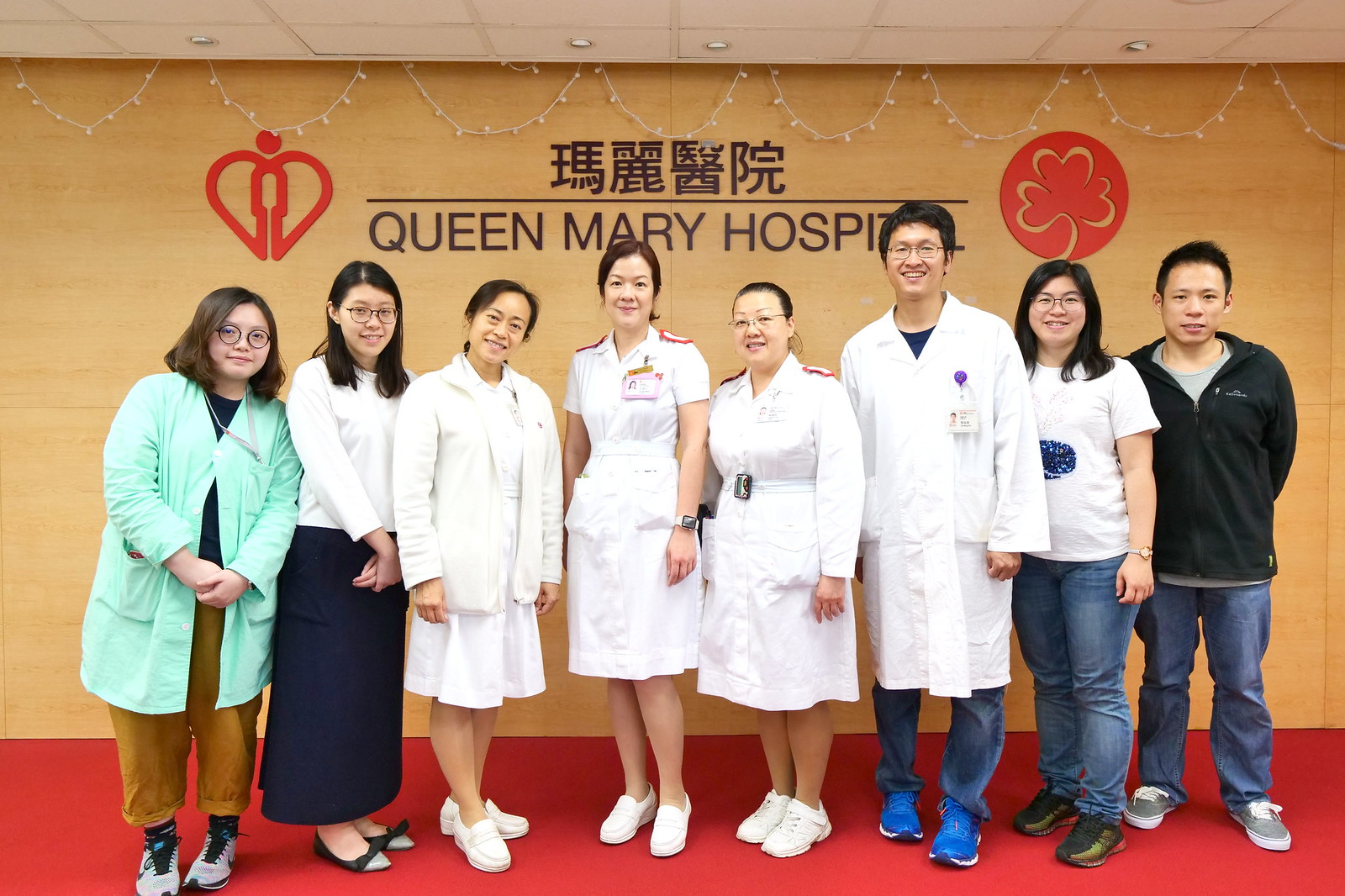In this detailed photograph, we see the diverse staff of Queen Mary Hospital standing against a golden yellow wall adorned with Chinese characters and black text that reads "Queen Mary Hospital." The background also features a heart logo on the left side and a shamrock logo encircled in red on the right. Eight medical professionals are lined up in front of the wall: six men and two women of varying roles and attire.

On the far left is a woman with short hair, glasses, and a smile, wearing a turquoise lab coat, mustard-colored pants, and athletic shoes. Next to her is another woman dressed in a white shirt and a navy dress, with shoulder-length hair and glasses. To her right stands an older woman in an all-white nurse uniform with white shoes, followed by another woman in a similar outfit but with glasses, indicative of their roles as nurses.

The next individual is a man in a doctor's lab coat that reaches his knees, desk badge on his left breast, jeans underneath, and blue shoes. Beside him stands a young woman with shoulder-length hair and glasses, dressed in a white t-shirt with an emblem, blue jeans, and black sneakers. Completing the group is a young man on the far right, wearing a black pullover top over a gray t-shirt, paired with blue jeans and gray sneakers.

They stand on a red floor, under a white ceiling adorned with inset bulbs and looped, unlit Christmas lights, contributing to a festive yet professional atmosphere. Judging by the bilingual signage, the setting could likely be in a Far Eastern region such as Hong Kong, lending an authentic cultural context to this vibrant and friendly group photograph.